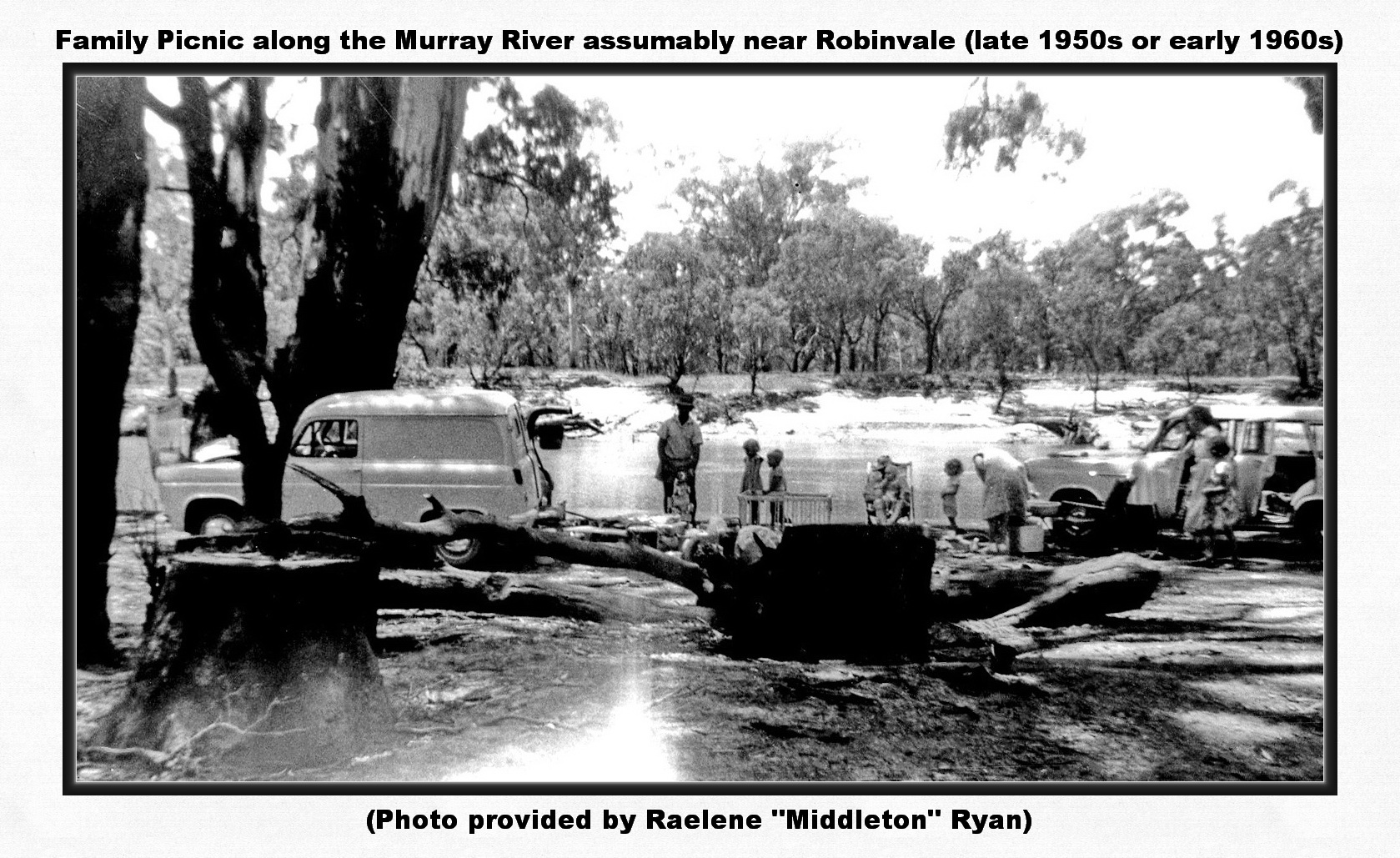The black and white photograph captures a nostalgic scene of a family picnic along the Murray River, presumably near Robinvale Lake, in the late 1950s or early 1960s. Two vintage cars are prominently parked, one being a panel truck with no back windows and the other a station wagon. A man stands at the open trunk of the panel truck, appearing to remove items. The scene is bustling with multiple adults and children; some are sitting on collapsible chairs, while others engage in conversation or stand beside a playpen where two younger children reside. Nearby, a child receives attention from a bending adult. The backdrop includes tall, leafy trees and a visible river, enhancing the picnic's serene natural setting. Notably, tree stumps are scattered in the foreground, indicating recent tree cutting. The photograph is framed with a silver or gray border, and the following caption is inscribed: “Family picnic along the Murray River, presumably near Robinvale, late 1950s or early 1960s. Photo provided by Rayling Middleton Ryan.”